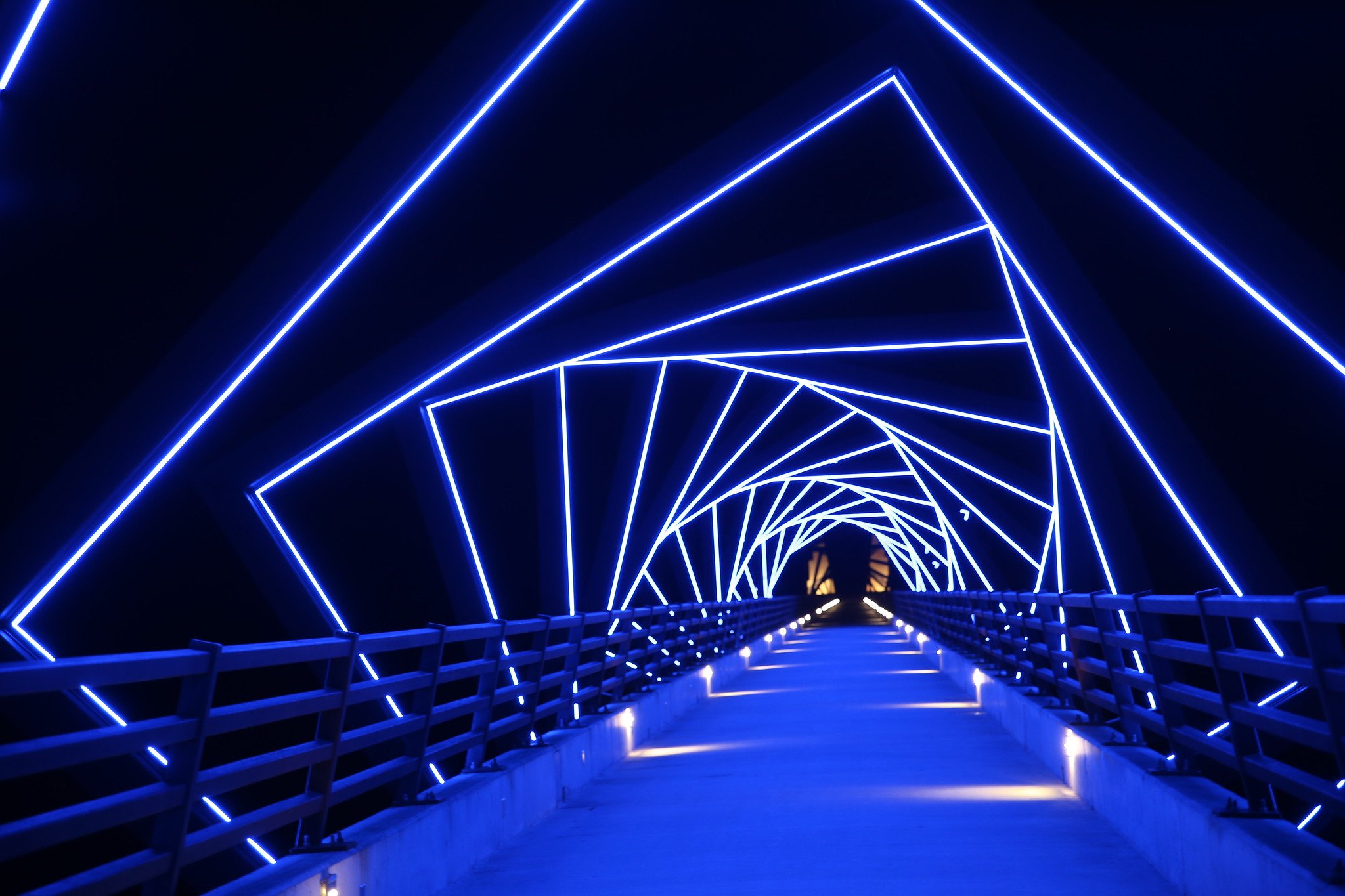The image depicts a futuristic, tunnel-like indoor bridge with a concrete pathway and metal side rails perched on a concrete base about half a foot to a foot tall. The scene is illuminated by a pattern of square lights that create geometric shapes along the pathway, extending straight ahead until it disappears into the darkness. These illuminated squares alternate between dark and light blue hues, giving the area a space-age appearance. The lighting creates a mesmerizing, slightly tilted tunnel effect, making the pathway appear as if it spirals gently. The ceiling of the structure is dark blue, while the edges of the squares glow brightly. Along the pathway, patches of light hint at smaller lights installed either along the bridge or emanating from the ceiling above. As the path extends into the night, a mysterious golden light at the far end casts a warm glow, with beams shooting upwards from either side, contrasting sharply with the surrounding blue hues and darkness.